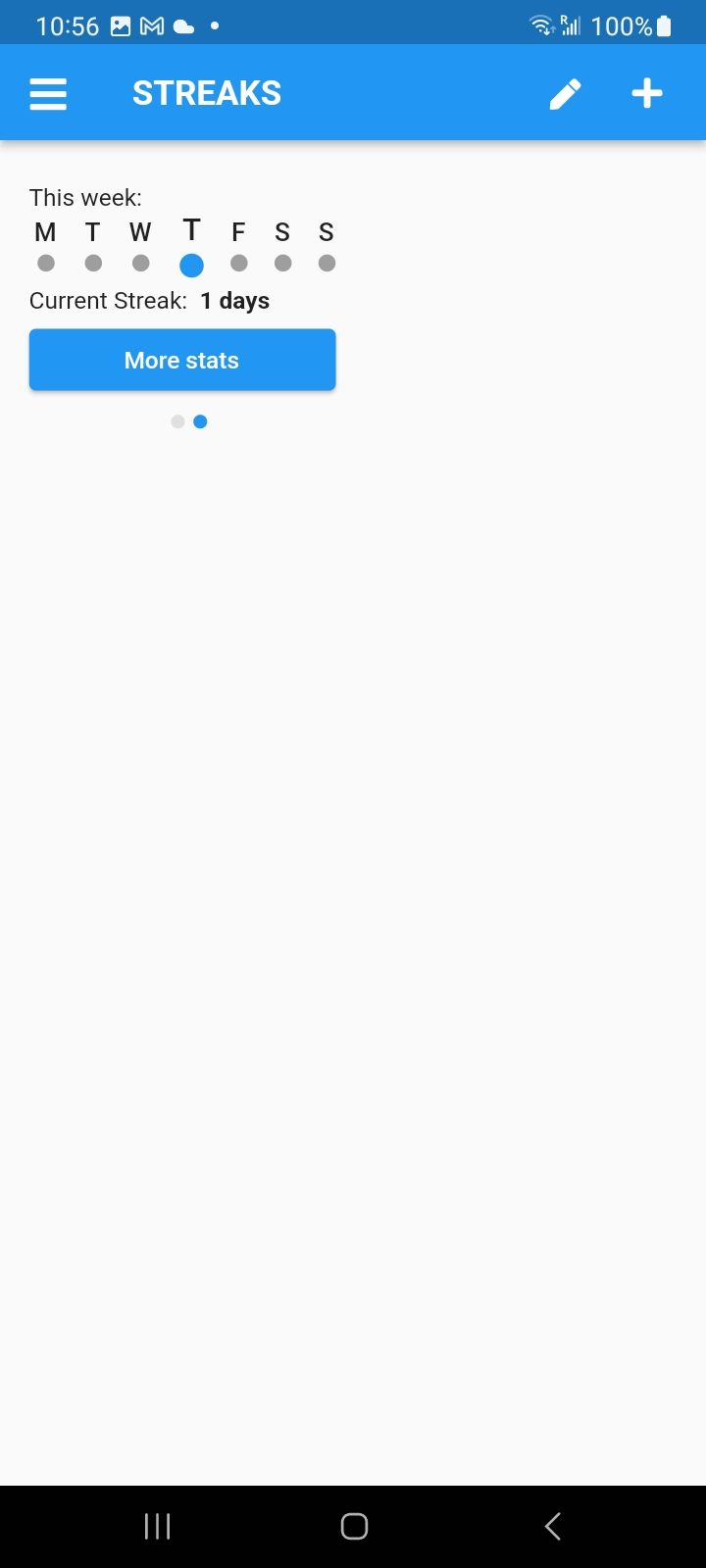The image depicts a cell phone screen with several distinct sections:

1. **Status Bar**: A dark blue strip at the top displaying:
   - The time "10:56"
   - Indicators such as "M" (possibly for notifications/messages)
   - A cloud icon
   - Data/Wi-Fi signal bars
   - Battery at 100%

2. **Header**:
   - A lighter blue strip just below the status bar
   - On the left, a menu icon comprising three horizontal lines
   - The word "STREAKS" in capital white letters
   - On the right, a pencil icon for editing and a plus sign

3. **Main Interface**:
   - A section with "This Week" written on a white background
   - Below that, the days of the week abbreviated as "M T W T F S S" in black letters, each inside gray circles
   - The "T" for Thursday has a blue circle beneath it, highlighting the current day
   - Below this, text stating "Current Streak: 1 day"
   - A "More Stats" button in white text on a blue background

4. **Indicator**:
   - Two small circles towards the bottom; the right circle is blue, indicating the current page, while the left circle is gray

5. **Bottom Navigation Bar**:
   - A black strip containing three horizontal bars next to each other, a circular icon, and a left-pointing arrow

**Color Scheme**:
   - Predominantly dark blue, lighter blue, white, black, and gray

The overall design suggests a focus on tracking some form of streak, although the specific type of streak (reading, fitness, diet, etc.) is not clearly identified.